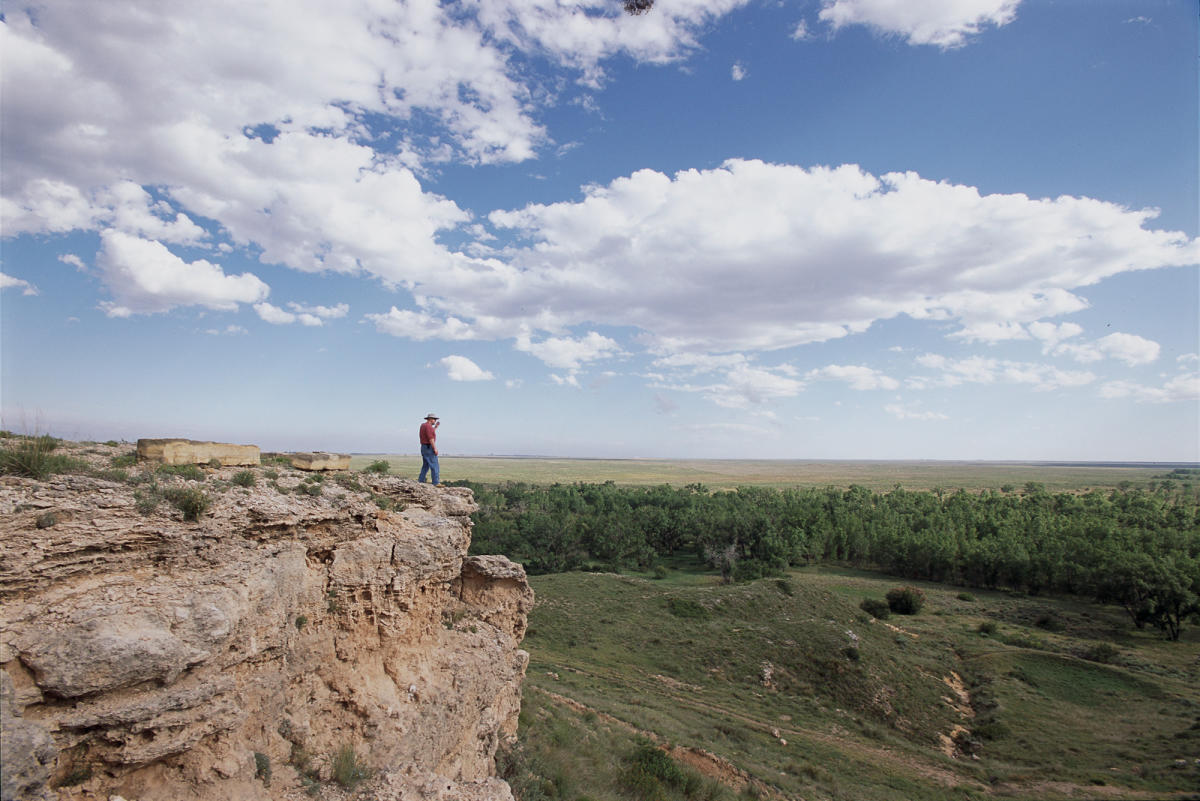In this daytime photograph, a picturesque scene unfolds under a vast blue sky filled with fluffy white clouds that fade to white near the horizon. Dominating the left side of the image is a tall, rugged cliff with a mixture of gray, whitish, tan, and even purplish hues interspersed with patches of green grass. Near the edge of this imposing cliff stands a man, distinct in his red shirt, blue jeans, and white hat, gazing down from the lofty height.

The landscape below extends into a large, uneven grassy plain punctuated by scattered hills and flat surfaces with tan and brown patches of earth. To the right, a sprawling green field with yellow accents stretches towards a line of dense trees that create a lush barrier. A couple of tan houses with brown rooftops can be seen in the distance, adding a touch of human presence to the otherwise natural scene.

In the far background on the right, a blue body of water glistens, reflecting the expansive, serene sky above. The overall composition captures the solitary figure at the cliff's edge, contemplating the wide, scenic expanse that unfolds before him, separated from the viewer by a significant, but visually bridging, gap.